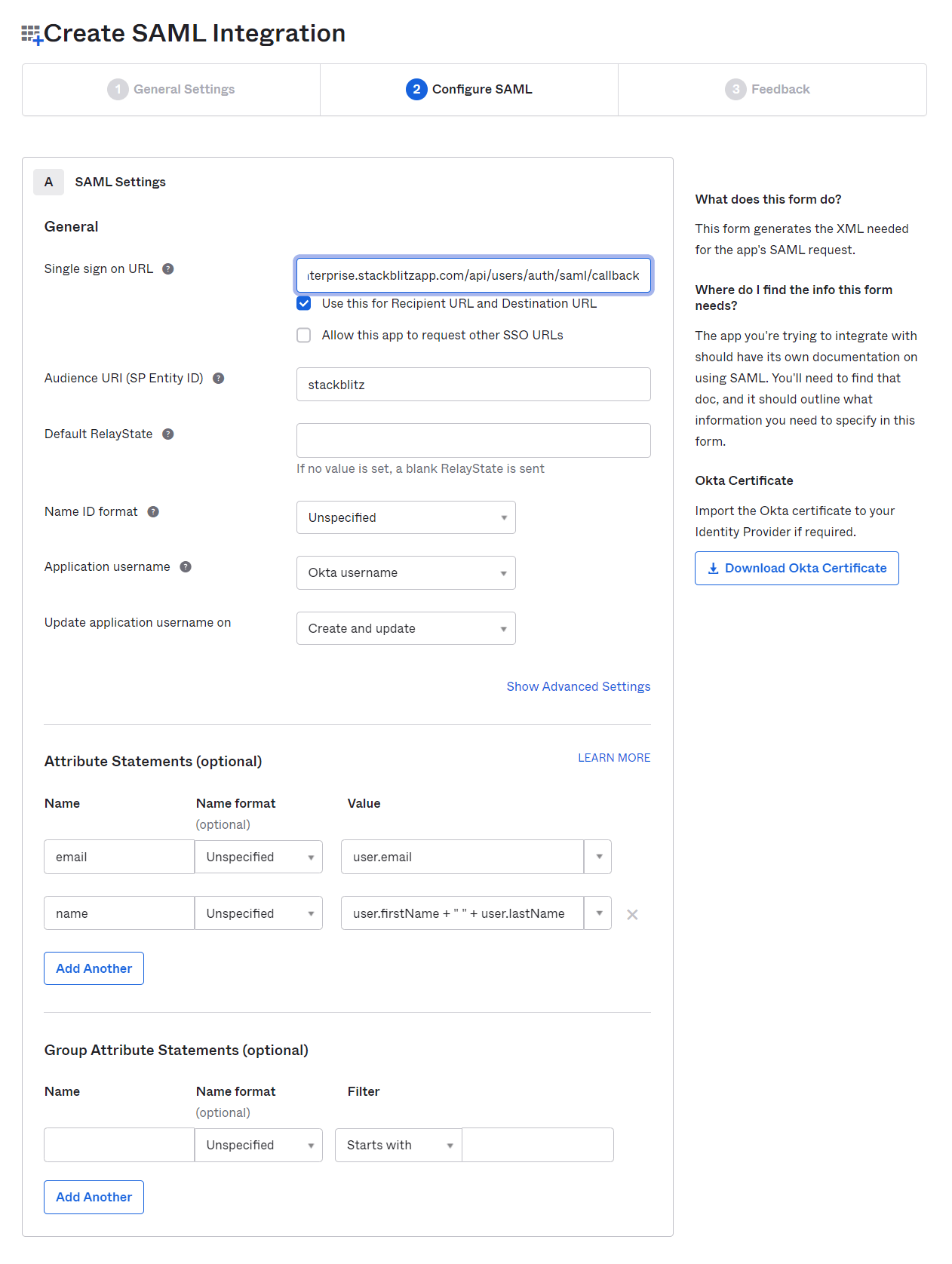Caption:
---
This screenshot features a web interface titled "Create SAML Integration." Positioned to the left of the title is an icon resembling a 3x3 grid of black squares, highlighted by a blue plus symbol at the bottom-right corner. Directly beneath the title, three menu tabs are displayed: "General Settings," marked by a gray circle with the number "1" but grayed out to indicate it is not selected; "Configure SAML," centered with a blue circle containing the number "2" and featuring bold black text to denote it as the active tab; and "Feedback," on the far right, featuring a gray circle with the number "3" in white inside, also grayed out to indicate it is not selected. 

The primary section of the page is structured for user input, divided into several subsections. The first subsection is labeled "SAML Settings," followed by "General Settings." Information fields are organized into two columns, with the left column providing descriptions accompanied by gray circles with question marks for additional help, and input boxes in the right column. The first row has a text entry box for the "Single Sign-On URL" and features two checkboxes underneath, with the first checkbox selected, labeled "Use this for recipient URL and destination URL."

There are five additional rows, with the first two containing text entry boxes and the last three comprising dropdown menus with unspecified options such as "Other Username" and "Create Updates." At the bottom-right of this section, there is an option to display advanced settings via a clickable box. 

Following a gray dividing line, the next section is "Attribute Statements," which offers more dropdown menus and an "Add Another" action button with blue text on a white background. Another dividing line leads to the "Group Attribute Statements" section, which similarly provides text entry boxes, dropdown menus, and an "Add Another" action button with a white background and blue text.

A secondary column, occupying approximately 20% of the page width on the right-hand side, provides informational content. It answers "What does this form do?" explaining that the form generates XML necessary for the app's SAML request. It also provides guidance on where to find the required information and offers a downloadable OKTA certificate via an action button featuring a download icon and blue "Download OKTA Certificate" text on a white background. This information occupies the top half of the column.

Overall, the interface is clearly segmented and user-friendly, guiding the user through the necessary steps to set up SAML integration efficiently.